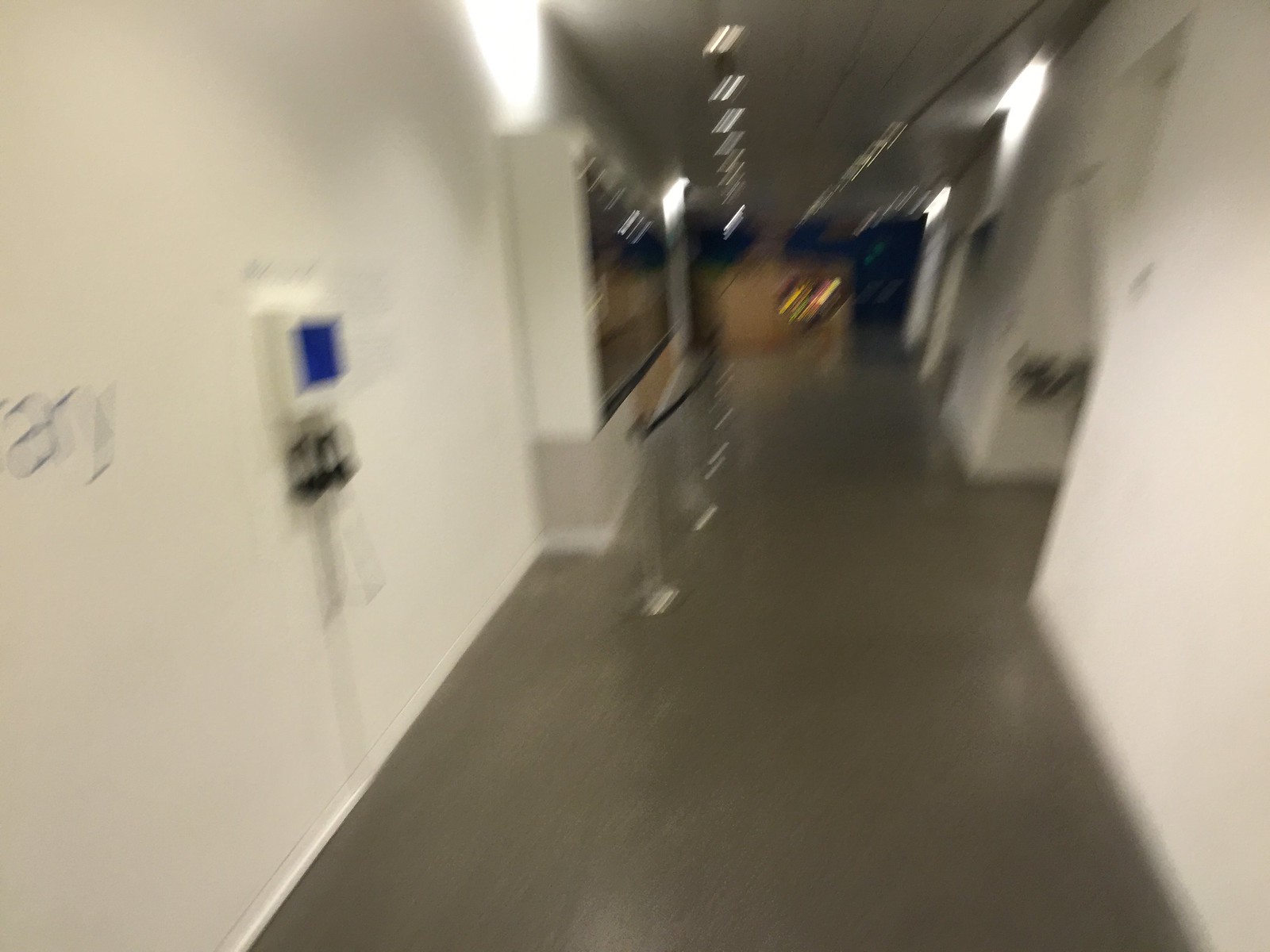The image depicts a blurry, out-of-focus indoor hallway with a shiny gray, likely concrete floor. The hallway stretches straight back from the viewpoint and is lined with white walls. On the left wall, there is a small, blue-screened item, possibly a thermostat, with two headphones hanging off it, hinting that it might be an interactive display often seen in museums. Next to this, there is some indistinct gray writing that is illegible. Farther down the hallway on the left side is a glass-fronted display case, though the contents are not visible due to the angle. In front of the case, there are silver-metal pedestal stands with black-banded strips preventing close access. The ceiling of the hallway features rows of hanging fluorescent lights that reflect off the shiny floor. Several hallways branch off to the right, but the image doesn't show what is down them, adding a sense of labyrinthine complexity to the space. The overall feel of the setting suggests it could be a museum, a gallery, or a luxury hotel.